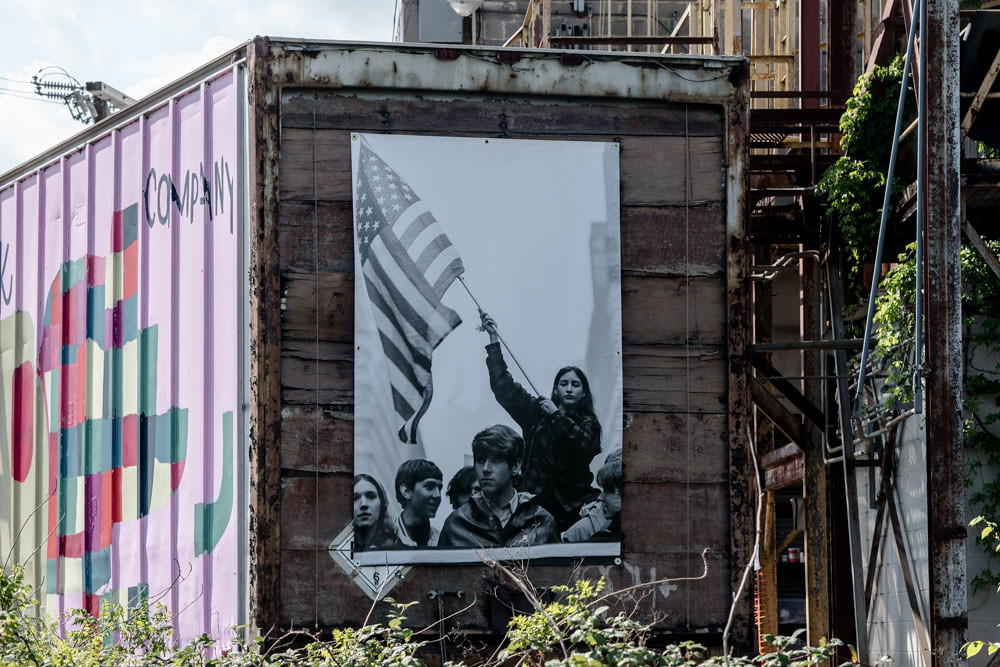In a sunlit photograph taken in the afternoon, an old and weathered train car, which might also be a semi-truck container, sits in a run-down urban area. The aged vehicle, largely constructed from decaying wood and painted white, features a large black-and-white poster pinned to its back. This poster depicts a group of young adults, possibly from the 1960s or early 70s, standing together in a city setting. Prominently, a teenage woman is elevated, possibly on someone's shoulders, holding and waving an American flag. Closer examination reveals a mix of emotions among the individuals, with some smiling while others appear serious. Below the poster, the sides of the vehicle are adorned with modern graffiti in vibrant colors including green, yellow, red, purple, and pink. The word "company" is spray-painted in black letters amid the eclectic designs. Adjacent to the container, rusty metal parts and construction debris contribute to the gritty ambiance. Overhead, the sky is a clear blue with minimal clouds, while a nearby building with a rusted fire escape and encroaching greenery adds to the scene's dilapidated charm.